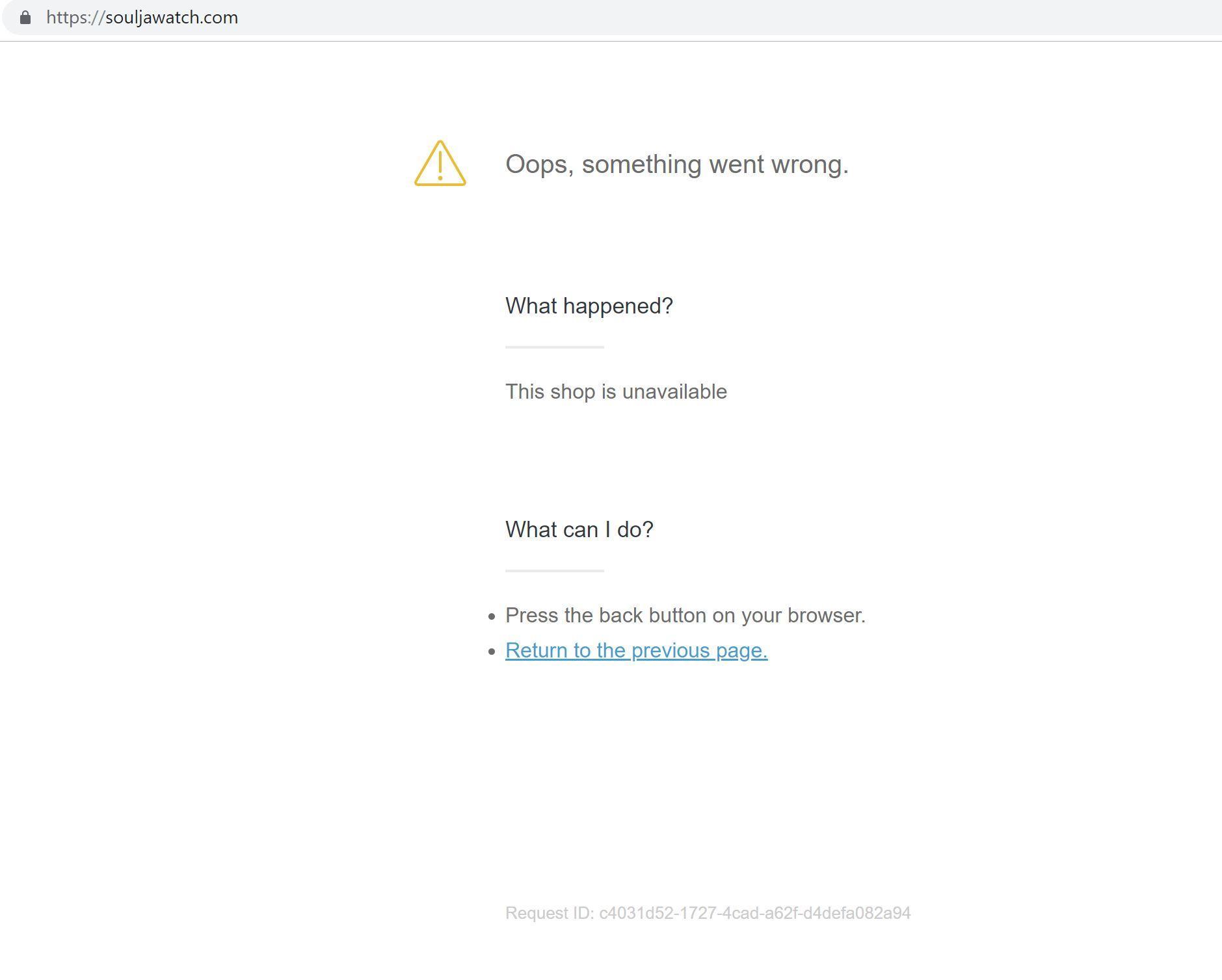A detailed caption of the screenshot could be:

"A screenshot of a webpage with a clean and minimalist design. The background is white, complemented by dark gray text. At the top of the page, the URL bar features a light gray background with a lock icon, indicating a secure connection, followed by the URL 'https://soldierwatch.com'. Beneath the URL bar, a thin gray line spans the width of the page. The main body of the page contains sparse text centered around a yellow triangle with an exclamation mark, indicating an error. Next to the triangle, the bold text reads, 'Oops, something went wrong.' Further down, a subheading inquires, 'What happened?' separated by another thin gray line. The subsequent text explains, 'This shop is unavailable.' Below this explanation, a considerable amount of blank space is followed by another inquiry, 'What can I do?' Beneath this question, another short, thin gray line precedes two bullet points: the first advises users to 'press the back button on your browser,' while the second, featuring blue underlined text, suggests users 'return to the previous page.' At the bottom of the page, light gray text provides a 'Request ID' followed by a unique string of letters, numbers, and dashes."